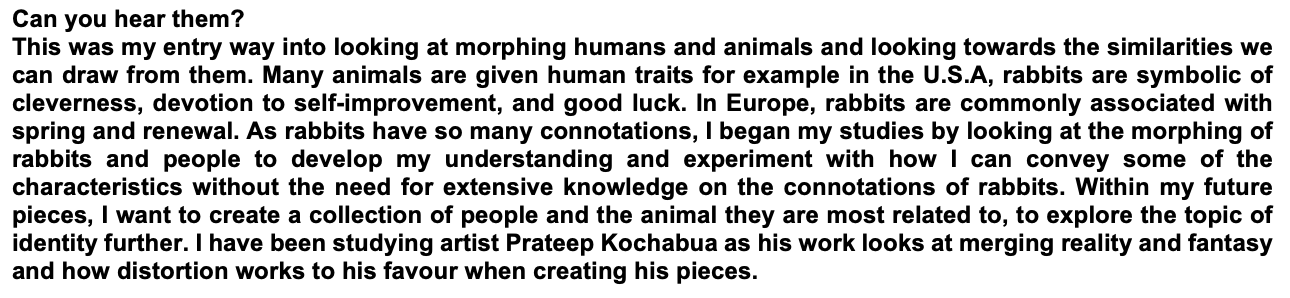The image depicts a landscape-oriented, justified paragraph of black text on a clean white background. The text begins with the question, "Can you hear them?" and continues to describe the author's entry into exploring the morphing of humans and animals, focusing on their shared characteristics. The author notes that many animals are imbued with human traits; for example, in the USA, rabbits symbolize cleverness, self-improvement, and good luck, while in Europe, they are associated with spring and renewal. The paragraph elaborates on the author's initial studies, which involved examining the morphing of rabbits and people to better understand and convey these characteristics without requiring extensive knowledge of rabbit connotations. The author expresses a future goal to create a collection exploring the identities of people and their animal counterparts. The text also references the artist Prateep Kochuboya, whose work merges reality with fantasy and leverages distortion to his advantage. The detailed and thoughtful typography underscores the conceptual depth of the study.